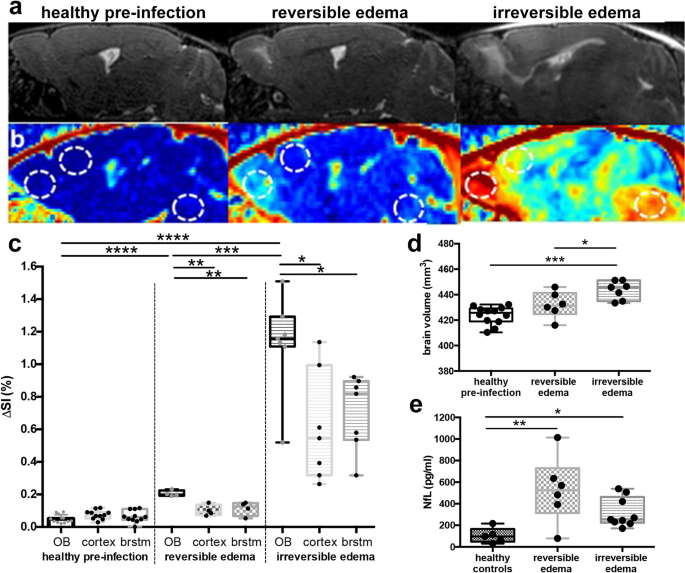The image is a scientific diagram composed of multiple panels, each focusing on different aspects of brain health and pathology. At the top, there are color-coded MRI scans, marked with A, B, and C, each showing various stages of brain conditions such as 'healthy pre-infection,' 'reversible edema,' and 'irreversible edema.' Notably, these MRIs have circles highlighting specific areas of interest. Below the MRIs, Panel B features thermal scans of the same conditions, also color-highlighted for emphasis.

Panel C provides detailed charts and explanations corresponding to the conditions depicted above, offering more technical information such as brain volume measurements and other relevant data points. Panels D and E include additional graphs and technical diagrams; D focuses on brain volume alterations, while E addresses NFL levels and the concepts of 'healthy controls,' 'reversible edema,' and 'irreversible edema.' This diagram is likely used for educational purposes, either to train medical students on how to interpret these scans or to guide doctors in diagnosing and treating the conditions discussed.